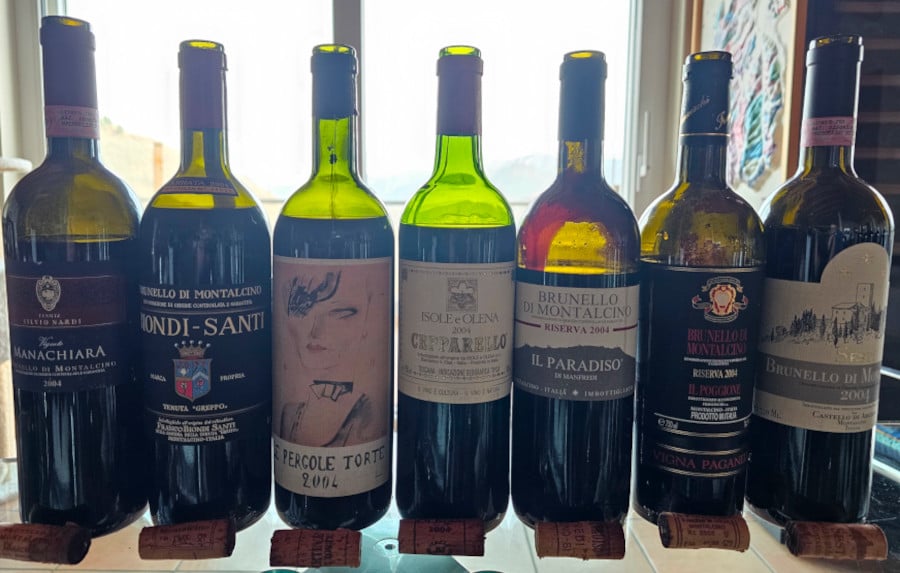This image shows seven elegantly labeled bottles of wine lined up side by side in front of a brightly lit window. Each bottle has its cork placed neatly in front of it on what appears to be a glass table or shelf. The labels are facing the viewer and include names like Manna Chiara, Bondi Santi, Percoi Torte 2004, Brunello di Montalcino, and Il Paradiso. The bottles are predominantly white wine, displayed in green glass. The background is washed out from the bright light outside the window, with a curtain visible on the right side and faint outlines of buildings. The close-up composition, with the careful arrangement of corks and vivid labels, possibly suggests someone's curated collection or a display, perhaps for a restaurant's menu.